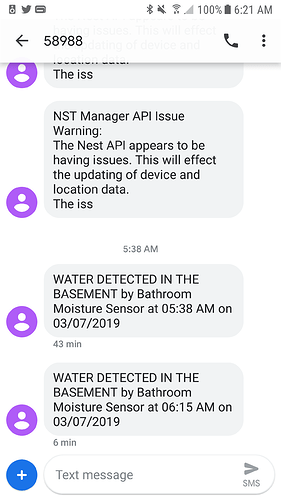A detailed screenshot of a smartphone's notifications panel is displayed against a white background. At the top left, there's a small square icon encompassing a circle, followed by a bird icon representing Twitter, and a folder icon. Moving to the right, a series of icons are aligned: a Bluetooth icon, a muted speaker indicator, a Wi-Fi signal, a cellular signal strength indicator, a battery percentage of 100%, and a battery icon.

In the middle, in black text, it reads "6:21 AM." Directly below this, aligned from left to right, there is a back arrow, an ID "58988," a telephone handset icon, and three vertical black dots.

Below this, there are three message notification bubbles. The first bubble is marked on the left with a little purple circle containing a white head-and-shoulders icon. The text inside this bubble reads: "NST Manager API Issue. Warning, the Nest API appears to be having issues. This will affect the updating of device and location data. The ISS."

In the middle of the notifications, it reads "5:38 AM." 

Below this, the second bubble states: "Water detected in the basement by bathroom moisture sensor at 5:38 AM on 3-7-2019." The time stamp to the left of this bubble shows "43 minutes."

The third bubble, also reporting an alert, states: "Water detected in the basement by bathroom moisture sensor at 6:15 AM on 3-7-2019." This is timestamped "6 minutes" to the left.

This descriptive caption provides a clear and structured overview of the key elements within the screenshot.